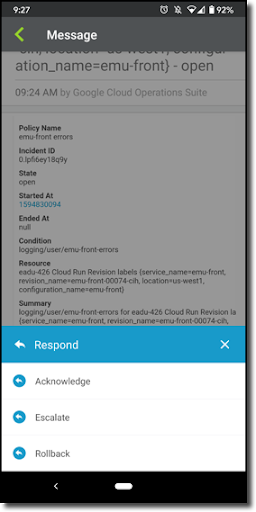This is an image of a cell phone screen displaying various interface elements. At the top of the screen, the time is shown as 9:27, and several icons are visible within a black upper bar. These icons include a shield, a notification bell (with one bell turned off and an active one), a clock, Wi-Fi signal strength, and a triangle. The battery indicator shows 92% with the battery icon filled in white.

Below this, there is a gray rectangle with a green arrow pointing to the right and the word "message" inside it. This area appears slightly grayed out due to an overlay popup box at the bottom. The bottom section of the screen features a bluish rectangle with the word "Respond" in white print, accompanied by an arrow pointing to the left and an "X" in the far right corner of the box.

Further down, there are options labeled "Acknowledge," "Escalate," and "Roll Back," each with a blue circle containing an arrow pointing to the left. The bottommost part of the screen displays a black rectangle with a leftward arrow and a small white line.